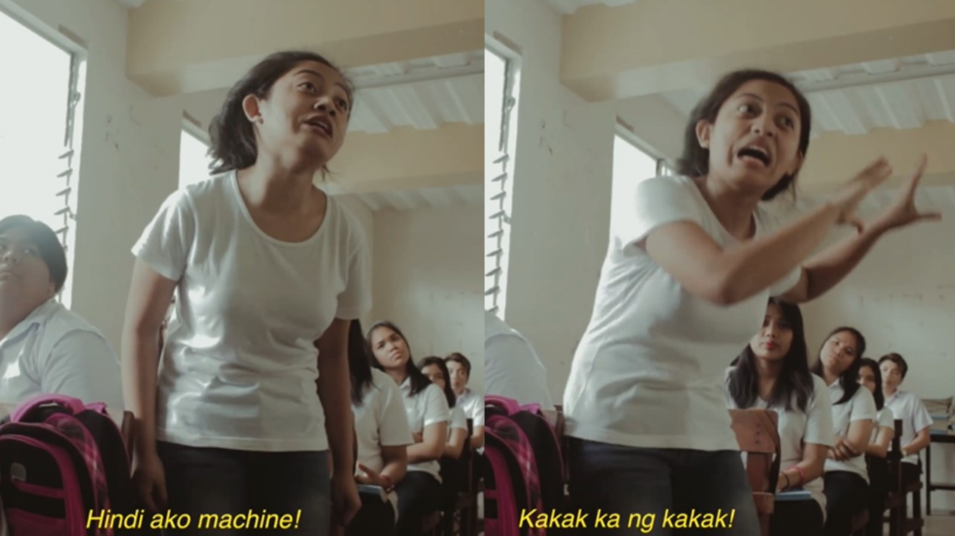The image depicts a classroom setting with two side-by-side photos of the same group of women, predominantly featuring a woman wearing a white scoop-neck t-shirt and dark pants. The room has off-white to yellow-toned walls, a tan ceiling, and two visible windows on the left side. Five women are seated in red chairs in both images, all dressed in white tops and dark pants. In the left photo, the woman stands in front of the seated group with a frustrated expression, her face contorted in a grin. Yellow text above her reads "Hindi Ako Machine!" In the right photo, she appears more animated, raising her hands with palms open as if yelling, while the text below reads "Kakak Ka Ng Kakak!" There are also red-checkered backpacks visible beside the woman. The overall scene captures a dramatic moment with distinct expressions and body language from the woman standing.